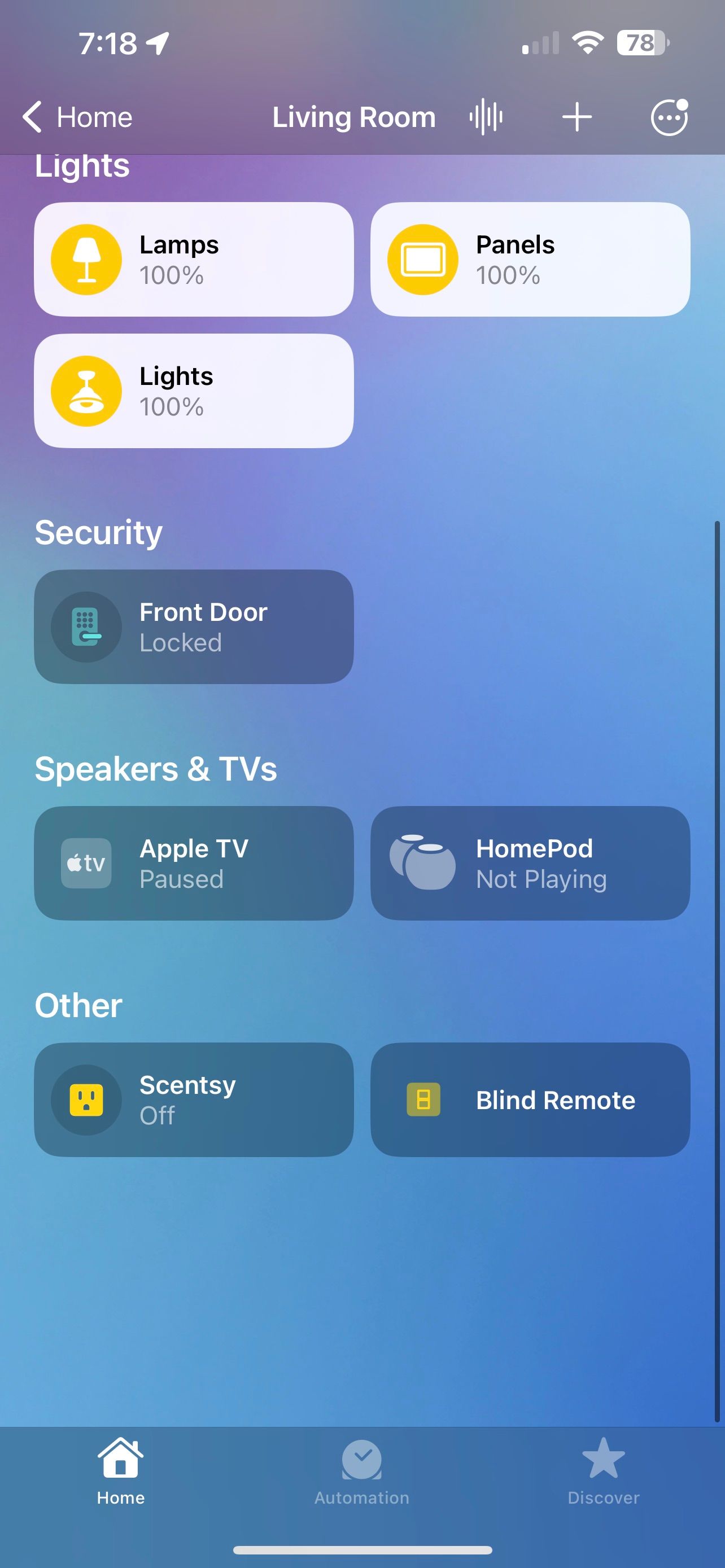The image showcases a cell phone screen in a vertical orientation, featuring a gradient background transitioning from purple at the top to blue at the bottom. At the top left corner, the time reads "7:18" alongside a small arrow pointing towards the 2 o'clock position. To the right, the status bar displays one out of four bars for cell phone signal strength, a full Wi-Fi indicator, and a battery icon showing 78%.

Directly below, a navigational toolbar includes a left-facing caret labeled "Home," with "Living Room" centered, followed by a series of vertical bars, a plus sign, and a circle with three dots. The section beneath, with a purple background, is titled "Lights" in white text. This section contains three control buttons for lighting: the first button labeled "Lamps, 100%" with a lamp icon, and next to it, "Panels, 100%" with a panel icon inside a yellow circle. Below these, the second button row includes "Lights, 100%" accompanied by a yellow circle and light icon.

Shifting towards the more blue-toned part of the screen, "Security" is written in white letters. A button below this is labeled "Front Door Locked." Continuing downward, the section titled "Speakers and TV" features two buttons: "Apple TV, paused" on the left and "HomePod, not playing" on the right. The "Other" section follows, containing two buttons labeled "Sensi, off" and "Blind Remote."

At the bottom of the screen, there are familiar cellphone navigation icons. The first icon, labeled "Home," is in white, while the next two options, "Automation" and "Discover," are grayed out.